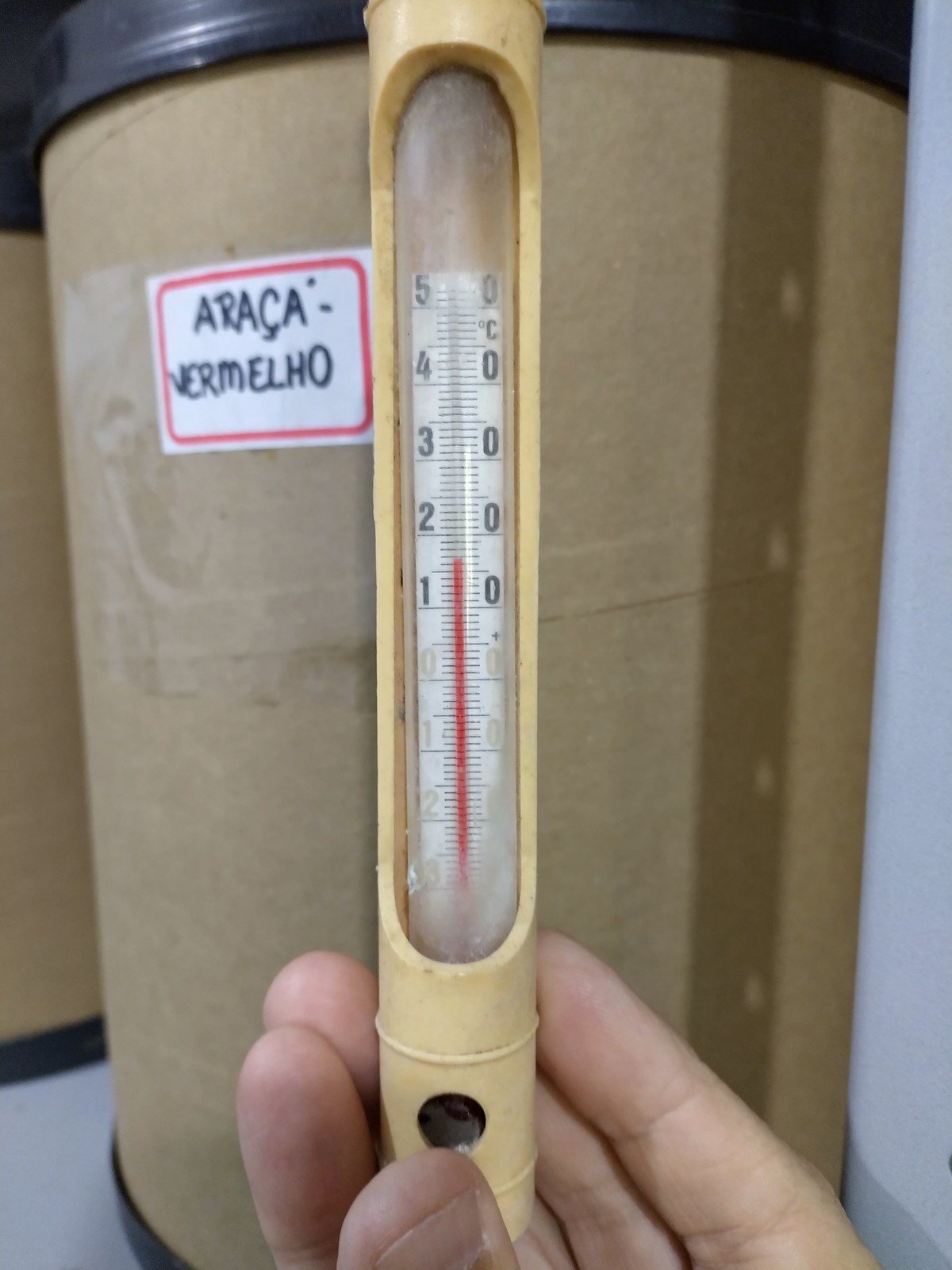In the image, a person is holding a pale yellow, tubular gauge with a clear plastic front cover, which reveals an inner mechanism resembling a thermometer. The gauge has numerical markings ranging from -3 to 5, with a red indicator line positioned just above the 1.5 mark. The background features a brown bin adorned with a white sticker outlined in red, displaying the text "Araca for Melho." The bin has a black top and bottom, providing a stark contrast to the more vibrant elements in the foreground.